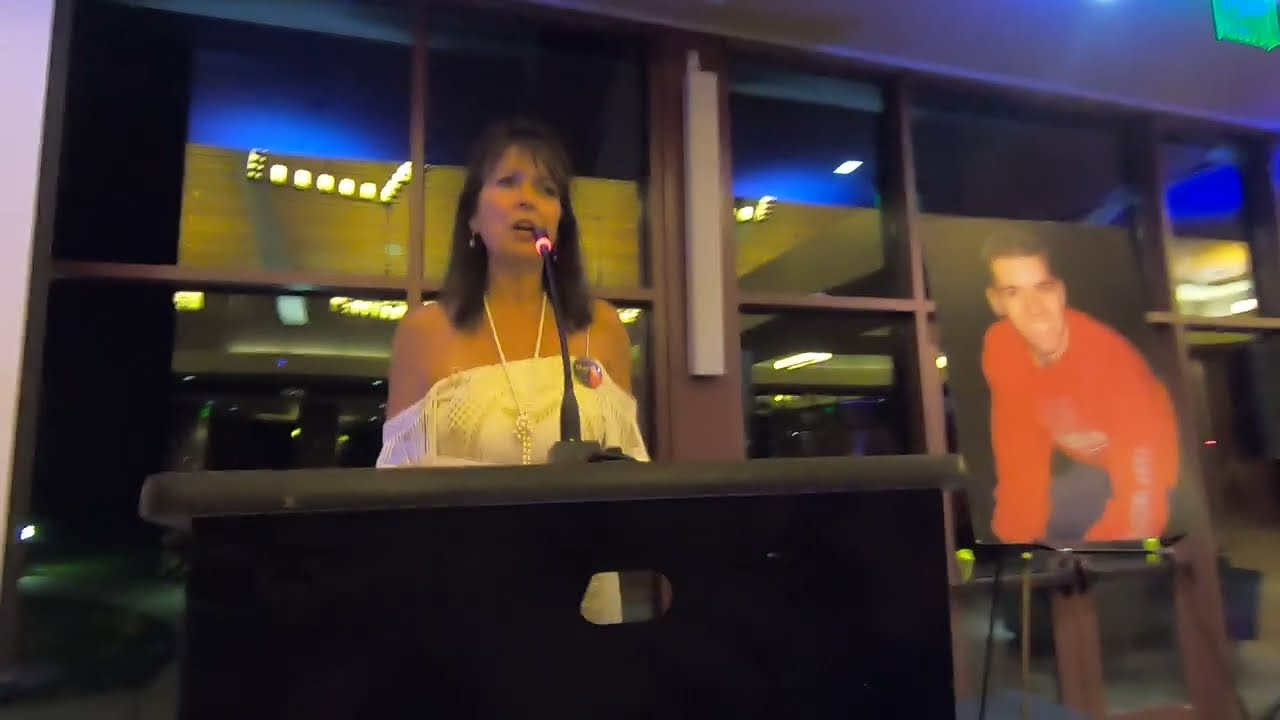In this image, a woman with shoulder-length black hair stands behind a sleek black podium, speaking into a thin black microphone adorned with a subtle red ring at the top. She is wearing an off-the-shoulder white top, accessorized with earrings and a pearl necklace, with a badge attached to her dress. The scene, filled with dark hues and hints of blue lighting, suggests it might be nighttime, as the large glass windows behind her are dark, reflecting ceiling lights. To the right of the podium is an easel holding a picture of a young man in a red long-sleeved shirt, smiling at the camera. Given the serious yet respectful atmosphere, it appears to be some sort of tribute or memorial event dedicated to him. The overall setting is indoors, with a blend of black, white, and red tones, along with minor green elements, contributing to the scene’s solemn ambiance.